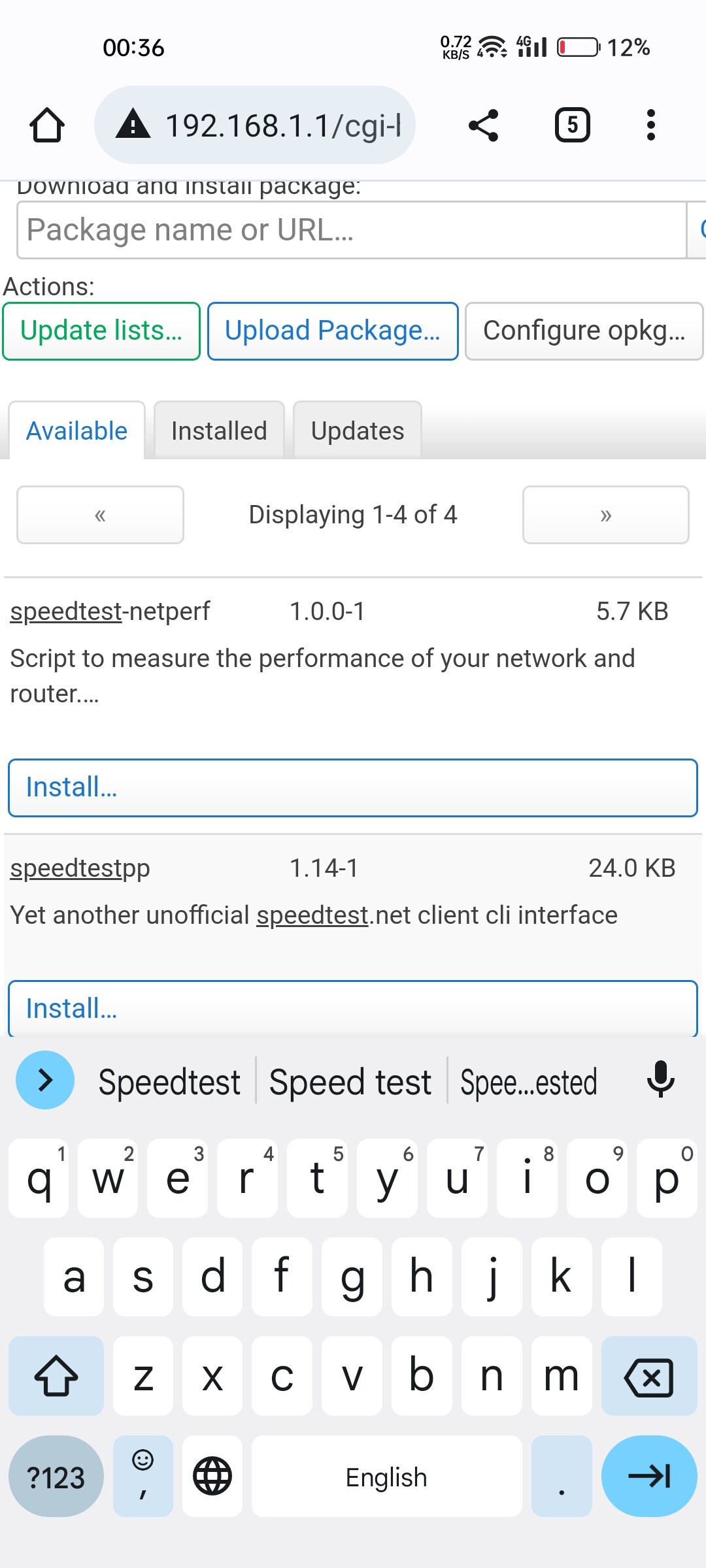This image is a detailed screenshot of a website interface displaying various system and network information and options.

At the top of the image, the time is shown as "00:36" in bold black text against a white background. To the right of the time, "0.72 KB/S" is displayed in all capital letters, indicating the current data speed. Adjacent to this, there is a WiFi signal icon, a "4G" symbol representing the cell signal strength, and a nearly depleted battery icon showing a red sliver with "12%" battery life remaining.

Below these icons, there is an image of a house symbolizing a homepage or home screen. Following this, an address bar appears with a gray background. Inside the address bar, there is a black triangle with an exclamation point, likely signaling a warning or error. The URL displayed is "192.168.1.1.1.1.1.1.cgi/l."

Further down, the text "Share" is positioned next to a square containing the number "5" and three vertical dots, possibly representing a share button and additional options menu.

The main content begins with the phrase "Download and Install Package," followed by placeholders for "Package Name or URL" and "Actions." Below this, there are several outlined blocks: a green one labeled "Update Lists," a blue one labeled "Upload Package," and a gray one labeled "Configure OPKG."

Next, there are three tabs: the first tab is white with blue text reading "Available," while the other two tabs are gray, labeled "Installed" and "Updates," respectively.

In the following section, a rectangular navigation bar features left and right arrows flanking the center text "Displaying 1.0.4.1.0.4.4."

Within the content area, the term "Speed Test" is prominently displayed, followed by details about two packages:

1. "Speed Test netperf 1.0.0-1 5.7 KB" with a descriptive note "Script to measure the performance of your network and router" and a button labeled "Install."
2. "Speed Test PP" underlined with the version "1.14-1 24.0 KB" noted as "Another unofficial SpeedTest.net client CLI interface," and marked as "Installed."

At the bottom of the image, a keyboard is partially visible, indicating that text input is possible or was recently used.